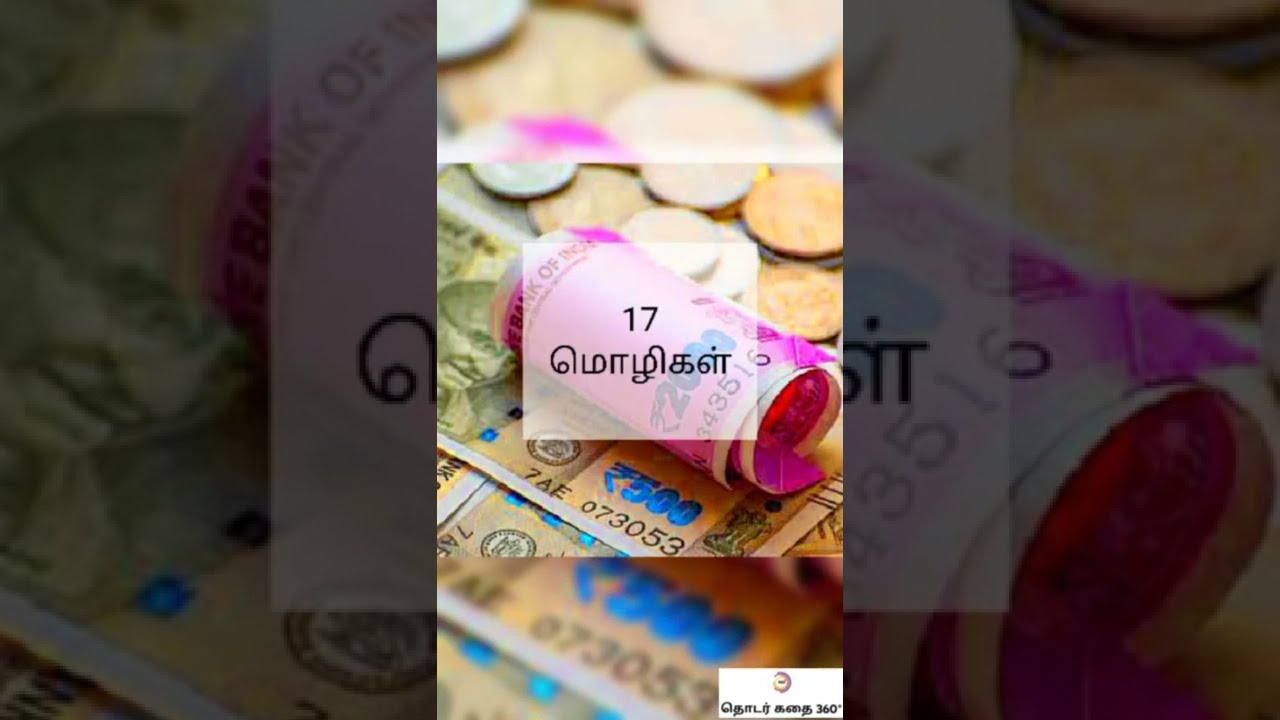The image showcases a collection of Indian currency, predominantly featuring various denominations of Indian rupees. In the center of the tall, rectangular frame, a tightly rolled 500-rupee note with a distinctive magenta hue takes prominence, flanked by several flat bills in shades of beige, blue, and green. Scattered around these paper notes are numerous silver and gold coins. Overlaying the currency, there's a semi-transparent black box displaying the number "17" along with some non-English text. The borders of the image are semi-transparent and blacked out but allow a glimpse of rupee notes, creating a framed effect around the central focus. Mahatma Gandhi’s face is discernible on one of the bills, emphasizing the Indian origin of the currency. The upper and lower parts of the photo are slightly blurred, directing attention towards the clear and detailed center, where the intricacies of the 500-rupee note can be observed.